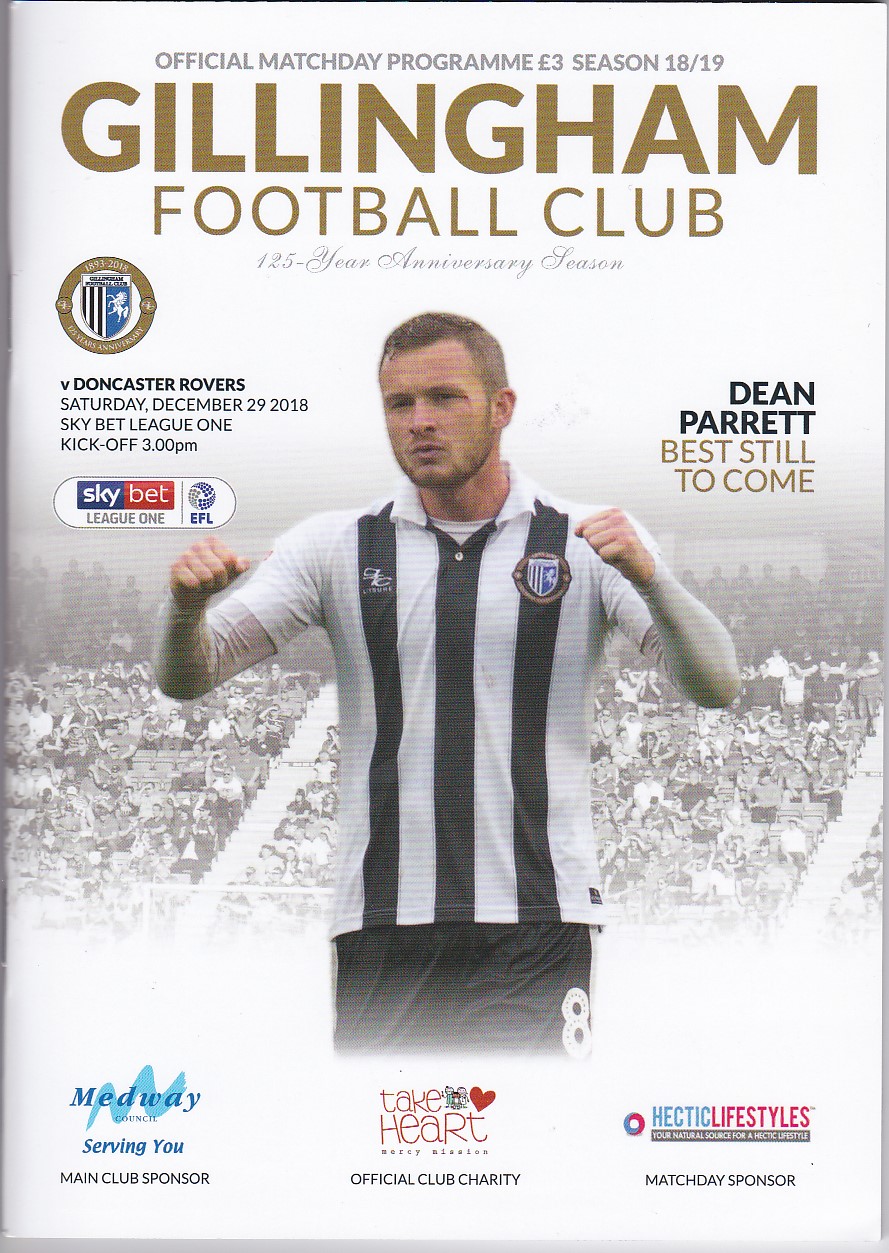The image is a cover of an official match day program for Gillingham Football Club's 125-year anniversary season. Dominating the center is a football player in a black and white striped top and black shorts with the number 8, celebrating against a black and white background of fans. The top header, written in gray letters, states "Official Match Day Program, £3.00, Season 18-19." Beneath this, "Gillingham Football Club" is rendered in gold font, accompanied by the text "125-year anniversary season" in smaller gray cursive. To the left, the club's circular shield logo is displayed, with "V. Doncaster Rovers, Saturday, December 29, 2018, Sky Bet League 1" and the kickoff time of 3 p.m. written below it. On the right, the text "Dean Parrett, best still to come" is prominently featured. The bottom portion includes various sponsor logos from left to right: Medway, Take Heart, and Hectic's Lifestyle. The color scheme includes shades of white, blue, black, red, pink, purple, gray, and gold, contributing to the dynamic and festive feel of the cover.